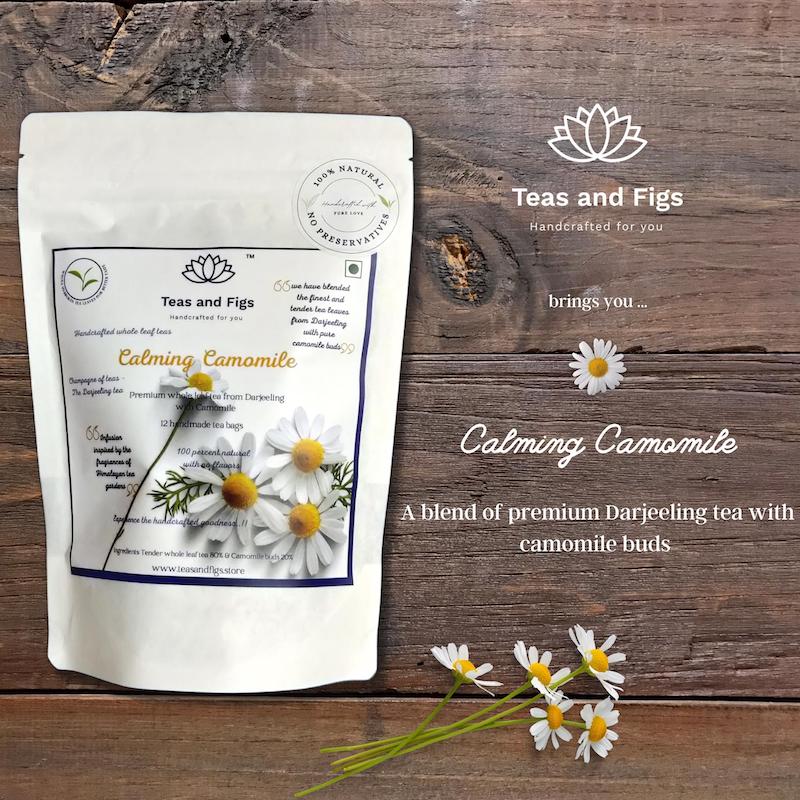In this visually captivating product photograph designed for a commercial setting such as an online shop or catalog, the focus is on a white bag of tea placed against a textured brown wood panel surface. The wood surface, detailed with dark brown and black knots and lines, consists of three horizontal planks, with noticeable wood knots in the upper left and central sections, enhancing the rustic aesthetic.

Occupying the left half of the image, the white tea bag prominently displays a large, intricate label. At the top right corner of the label, within a circular emblem, it boldly reads "100% Natural, No Preservatives." The label, adorned with delicate illustrations of white flowers resembling daisies or carnations, declares "Teas and Figs" in black text. Below the main title, in elegant yellow cursive, it states "Calming Chamomile." Further textual details elaborating on the product include "Handcrafted for You" and "Premium White Tea from Darjeeling," emphasizing the artisanal and high-quality nature of the tea. The package contains "12 Handmade Tea Bags," making it an inviting choice for consumers seeking a calming, natural tea experience.